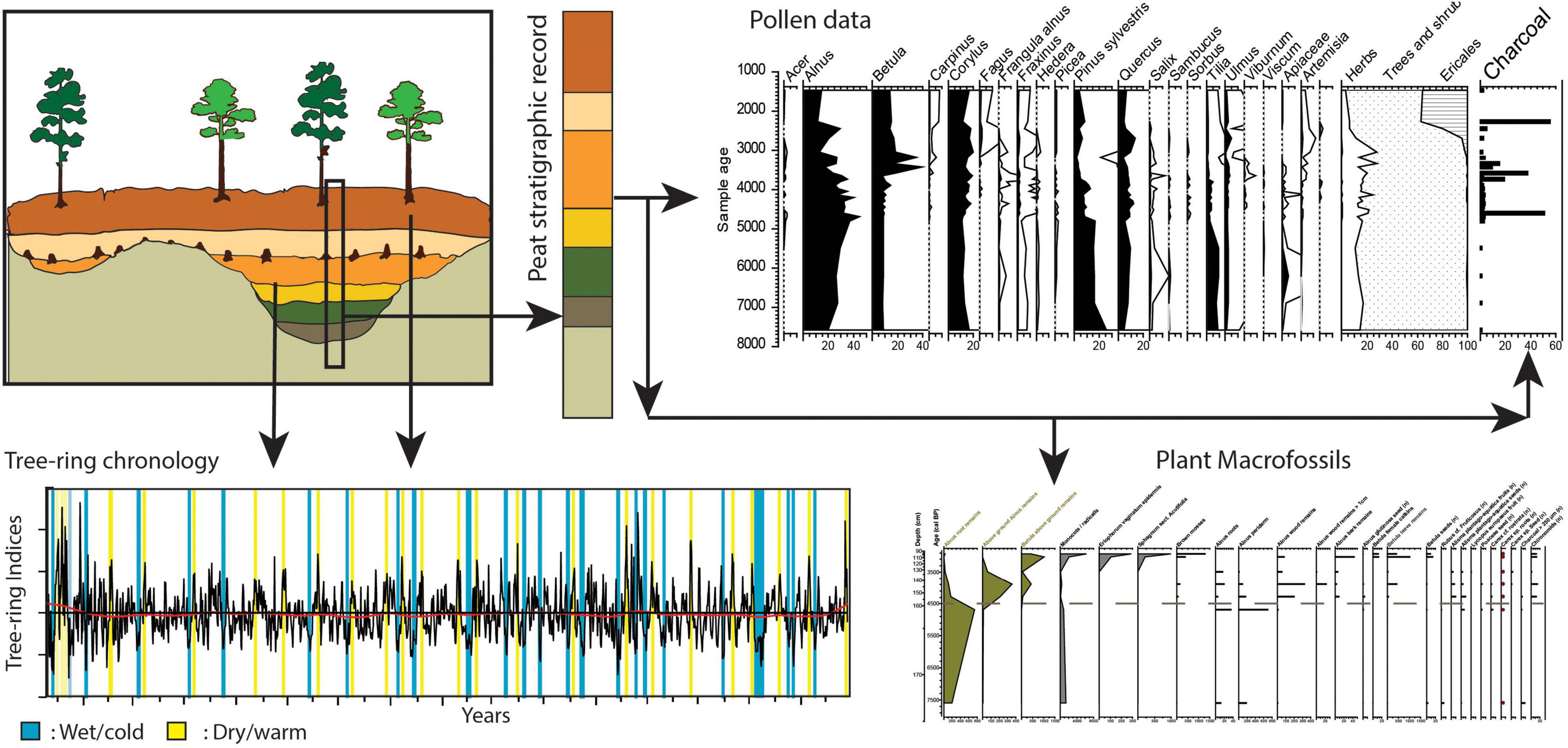The image is a horizontally oriented rectangular infographic with a white background, divided into multiple sections with a series of detailed illustrations and graphs. 

In the top left corner, there's an illustrated cross-section of soil showing its stratigraphic layers. The layers start with a dark brown topsoil, followed by light brown, orange, yellow, green, and gray layers. On the surface, four trees alternate in color from dark green to light green from left to right. Beside this illustration, an up-and-down bar indicates the different soil types.

To the right of the soil illustration is a segment labeled "Pollen Data," which contains a graph depicting the pollen quantity from various plants over time. 

Beneath this segment is another labeled "Tree Ring Chronology," featuring graphs with black markings on a white background, resembling heart rate monitors. These graphs include blue and yellow bars indicating climatic conditions, where blue represents wet and cold, and yellow signifies dry and warm periods. 

The bottom right section of the infographic is dedicated to "Plant Microfossils." This section features a graph with lines that create small sections, each containing data about different microfossils.

Arrows and labels throughout the image guide the viewer through the various data presentations, highlighting the complex relationships between soil layers, pollen data, tree ring chronology, and plant microfossils.